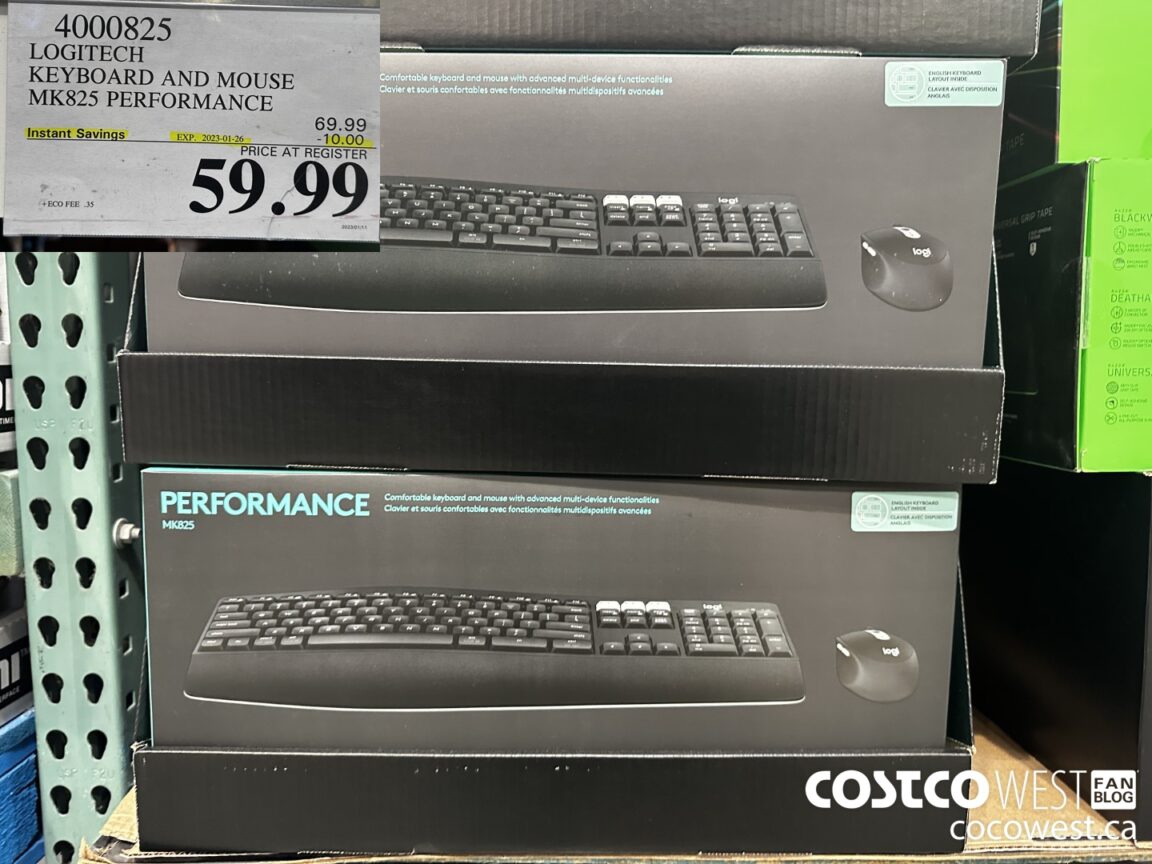The photograph captures a neatly organized retail display of Logitech keyboard and mouse sets on a shelf. In the upper left-hand corner, there's a partially cropped white rectangle with the bold black numbers "4000825" visible at the bottom. Below that, the bold, uppercase text "LOGITECH" is prominently displayed, followed by the product name "Keyboard and Mouse" and model information "MK825 Performance" in a smaller font. 

In the lower right-hand corner of this white rectangle is the price, clearly marked in large bold numerals: "$59.99". The edge of the green metal shelf, which features black adjustment holes, is visible running down the left side of the image.

To the right of the green shelf edge are two gray display boxes, which contain the product packaging. Each black box features "PERFORMANCE" in blue-green all caps at the top left, with two lines of small text in the same color to the right. In the upper right-hand corner of each box, a light green rectangle contains additional black text. 

Centrally, at the bottom of each box, there is an image of a black keyboard shot from a top-down angle, showing the back of the device. To the right of the keyboard, a black mouse with light gray buttons and a rollerball is depicted. This keyboard-and-mouse image is repeated once more on the display.